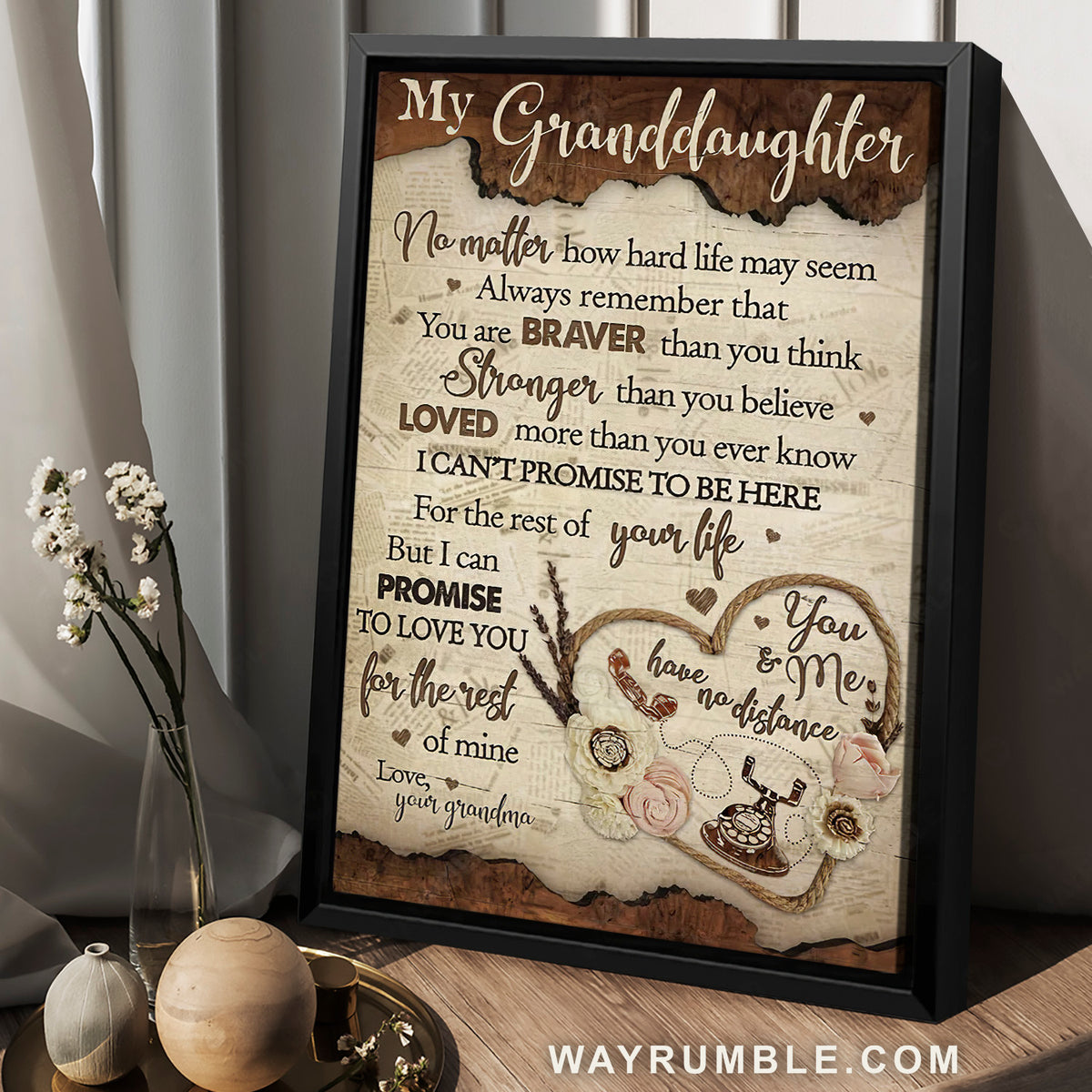The image features a charming art print with a black frame, set against a white curtain or textured wall. The print, which rests on a rustic wooden table, bears a heartfelt message from a grandmother to her granddaughter. The message reads, "My granddaughter, no matter how hard life may seem, always remember that you are braver than you think, stronger than you believe, and loved more than you could ever know. I can't promise to be here for the rest of your life, but I can promise to love you for the rest of mine. Love, your grandma." The background of the print is dark brown at the top with white text, and beige in the lower part with brown text. Accent elements including a heart made from rope and an antique rotary phone illustration add to its sentimental value. The print sits alongside a small tray with decorative items, a clear glass vase with fresh white flowers, and other small vases. At the bottom of the picture, the website "WayRumble.com" is prominently displayed in bold, all-uppercase white letters.